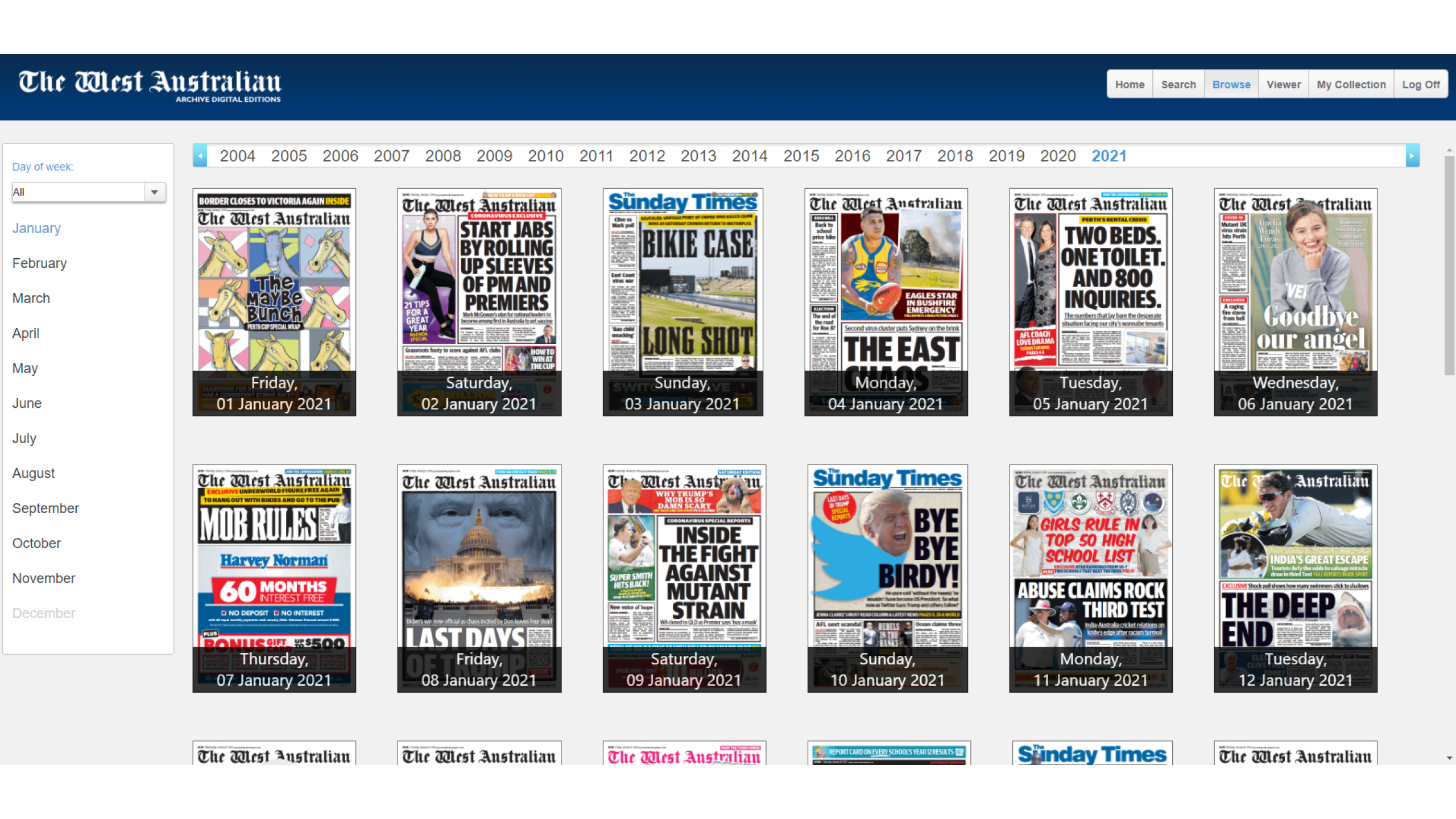Screenshot of a webpage from "The West Australian" website. The top of the page features the site’s logo in elegant calligraphy against a blue background. Below the logo, the heading reads "Achieve Digital Editions." The main section displays a list of years from 2004 to 2021, with 2021 highlighted in blue, indicating it has been selected. The page includes numerous articles from "The West Australian" and features content from "The Sunday Times" as well. There are a total of twelve clickable items organized in two rows, with six in each row, providing navigation options for additional content.